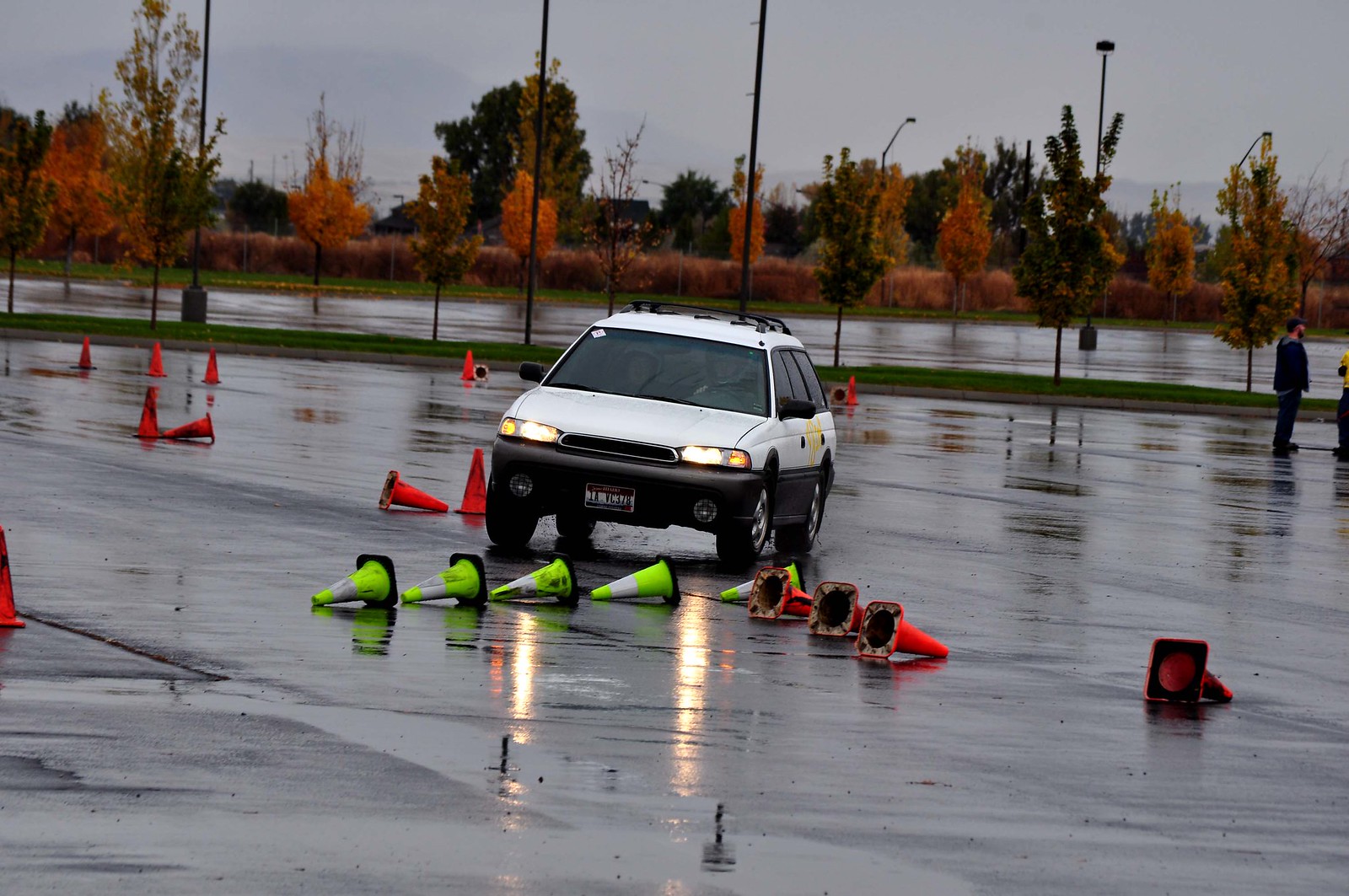The image depicts an outdoor, daytime scene in a large, wet parking lot, suggesting recent or ongoing rainfall. Centered in the photograph, a small, older-model white four-door hatchback is navigating a course outlined by a mix of orange and fluorescent green street cones. The car is captured in a three-quarter view from the front left, with its headlights on, and appears to be tilting slightly to the right, indicating a hard right turn. Many cones are knocked over, possibly due to the weather, as there is no evidence of the car making contact with them. In the background, the trees and shrubs display vibrant fall colors, ranging from yellows to oranges, further emphasizing the season. Additionally, two men are seen conversing to the top right of the frame, suggesting the presence of driving instructors supervising the course.